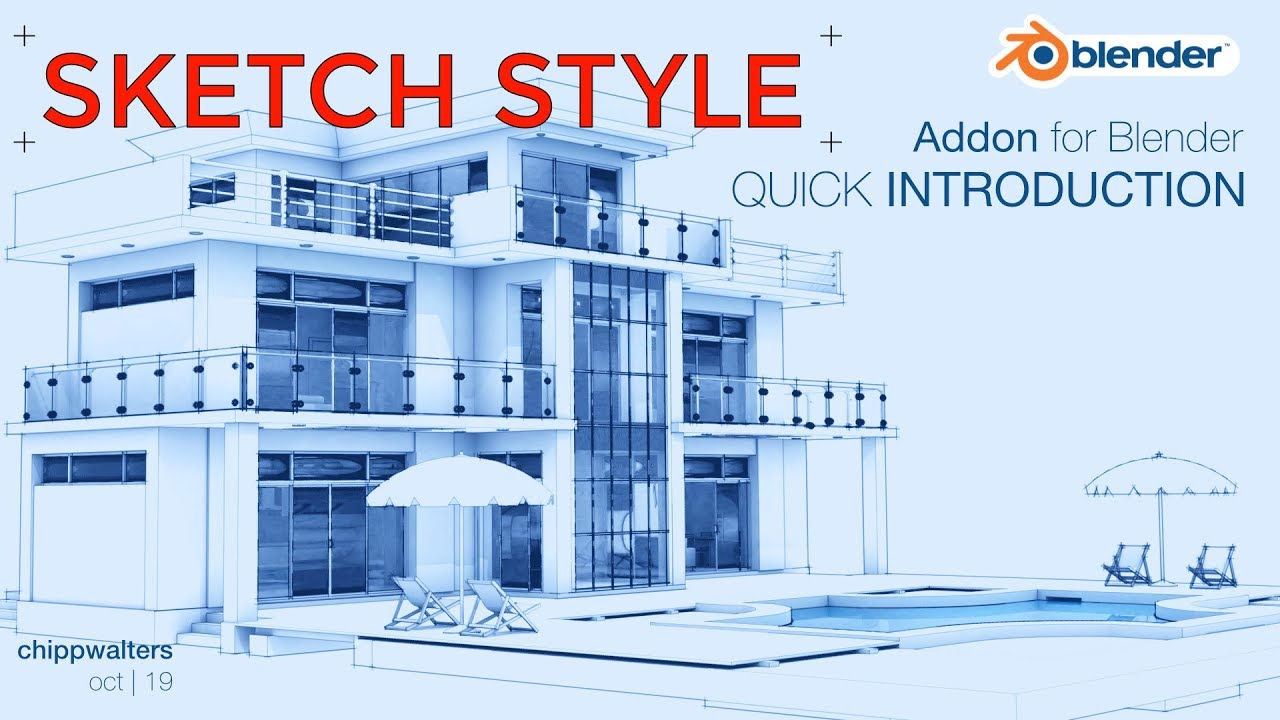This infographic features a light blue background and showcases a detailed digital semi-sketch style rendering of a modern multi-story building. The building is characterized by its large glass windows and balconies with sleek glass railings. In the foreground, there is a pool area accompanied by two umbrellas and several lawn chairs, providing a sense of luxury and relaxation. Highlighted in red text, the graphic proclaims "Sketch Style," with blue text below it stating "Addon for Blender, Quick Introduction." At the bottom of the infographic, the creator's name, "Chip Walters," along with the date, "October 19," is clearly displayed. Additionally, the top corner features the official Blender logo, which includes an orange swirl design with a blue dot.